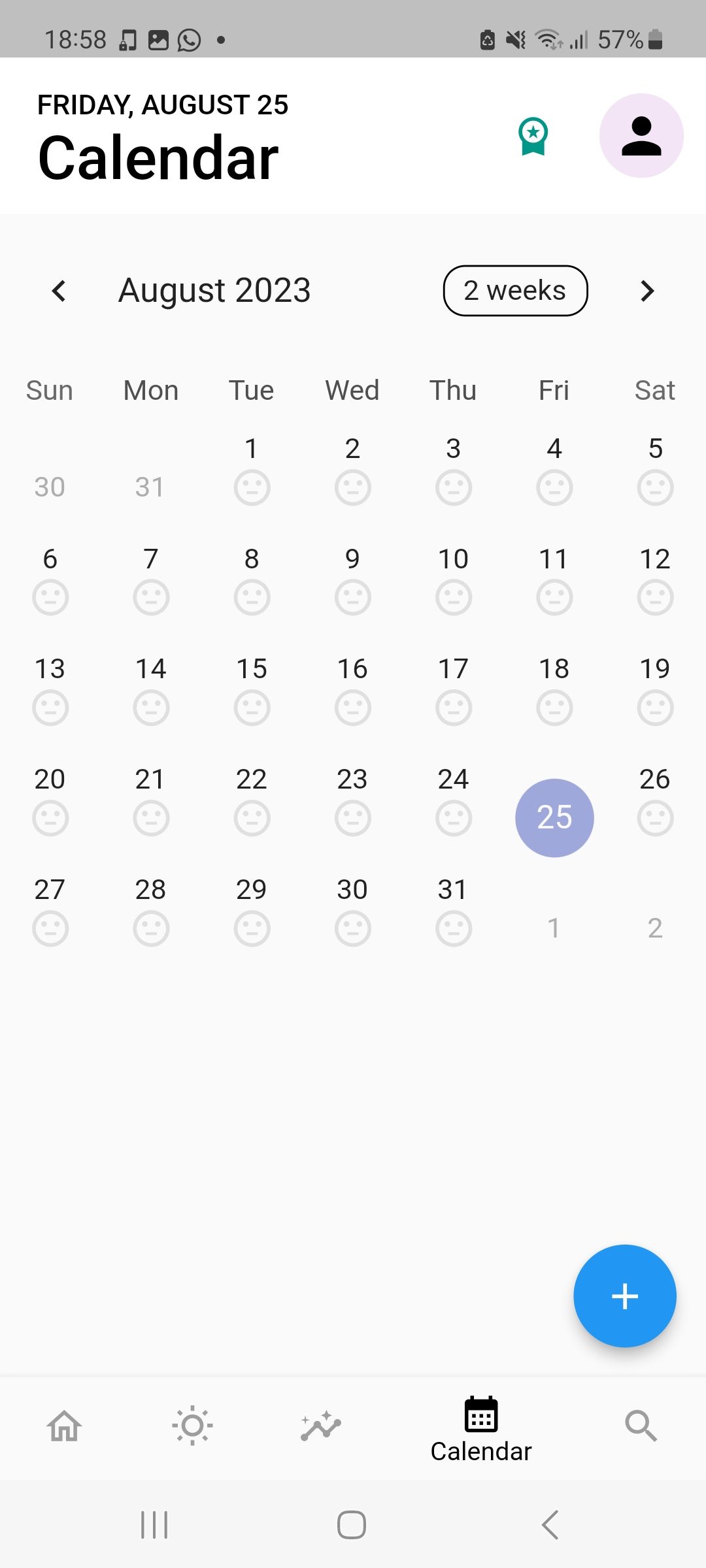The image depicts an iPhone screen displaying a calendar app. The phone's battery life is at 57%, indicating that it is adequately charged. The status bar also shows that the sound is turned off, and the current time is 18:58 (6:58 PM). It is Friday, August 25th.

The calendar application interface prominently features the word "Calendar" at the top. Beneath it, "Friday, August 25th" is displayed in slightly smaller text. Just above the calendar grid, there is an icon resembling a circle on a base with a green star inside it, against a white background.

Adjacent to this icon is a generic profile picture represented by a pink circle with a simplistic human silhouette. The calendar grid features a very light gray background, marked as "August 2023" on the left side and "Two Weeks" circled on the right side.

The days of the week are listed horizontally: Sunday, Monday, Tuesday, Wednesday, Thursday, Friday, and Saturday. The dates start on Tuesday the first and continue sequentially. Notably, the dates bear small face icons under them, all of which have neutral or sad expressions, indicated by downturned mouths.

The date "Friday, August 25th" is distinctly marked with a blue circle around it. At the bottom of the calendar interface, there is a plus sign (+) in a lighter blue color, which suggests an option to add new events or reminders. Additionally, there are icons at the very bottom for navigation—home, calendar, search, and two other unspecified icons.